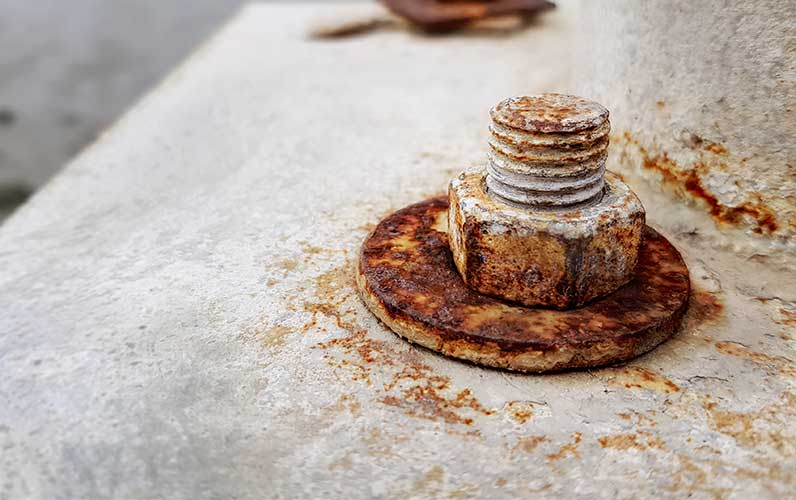The image showcases a rusted screw, washer, and bolt assembly prominently set against a plain, gray surface. Starting from the bottom, the washer is in direct contact with the surface, displaying heavy rust with dark brown and black spots throughout. Above the washer is the bolt, retaining some of its original gray hue but with significant rust on its outer edges. The screw, visible at the top, maintains some silvery color but also shows patches of rust. The gray surface underneath the hardware also features patches of rust around the washer area. The background of the image is blurred, with a dark gray section in the upper left, and another rust-colored object in the upper center. Overall, the scene conveys a sense of decay and oxidation.